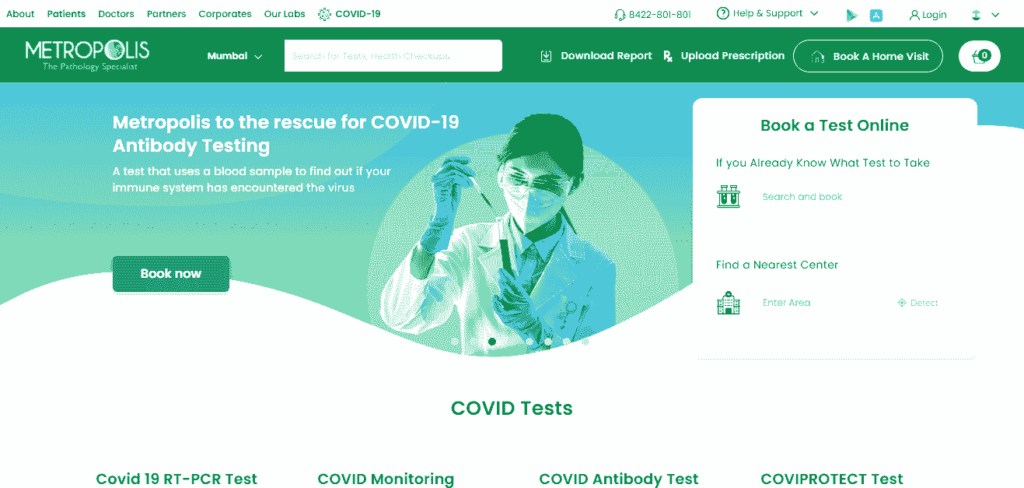This is a detailed screenshot from a computer displaying the Metropolis website homepage. 

**Top Navigation Bar:**
- The background is white with green text. From left to right, the navigation options include: About, Patients, Doctors, Partners, Corporates, Our Labs. 
- An icon followed by "COVID-19" is situated toward the middle-right.
- Just right of center, there's a headphone icon next to the contact number "8422-801-801."
- Following is a green-outlined circle with a green question mark labeled "Help & Support" which features a dropdown arrow.
- The Google Play Store icon, represented by a white 'A' in a teal square, appears next.
- Followed by a profile icon and the word "Login."
- To the far right, there are an up arrow with a line under it and a dropdown arrow.

**Header Bar:**
- A dark green bar features "METROPOLIS" in all-capital white letters. The second 'O' in "METROPOLIS" contains an indiscernible image.
- Below in smaller white letters: "The Pathology Specialist."
- To the right, "MUMBAL" with a dropdown arrow.
- A white search box follows.
- Then, a download icon and "Download Report."
- An RX icon with "Upload Prescription."
- A white outline oval icon with a house and "Book a Home Visit."
- A white oval icon with a shopping basket featuring a green circle and '0' indicating the cart status.

**Main Section:**
- Background transitions from blue to green in a wavy pattern.
- The top of a white box cut into this background features a doctor in protective gear (gloves, face mask, and glasses), hair pulled back, in a white jacket. The doctor is using a syringe to add fluid to an already two-thirds-full test tube.
- Text within this white box:
  - Metropolis' slogan: "Metropolis to the rescue for COVID-19 antibody testing."
  - Smaller text below: "A test that uses a blood sample to find out if your immune system has encountered the virus."
  - A green box at the bottom with "Book Now" in white text.

**Booking Section:**
- Within the white box:
  - Green text: "Book a test online" (bold) followed by: "If you already know what test to take."
  - Icon with two test tubes and "Search & Book."
- Another option: "Find a Nearest Center" with an icon resembling a hospital building, followed by "Enter Area."

**Footer Section:**
- Light green line separating sections.
- Bold green header: "COVID Tests"
  - Subsections in smaller bold green text: 
    - "COVID-19 RT-PCR Test"
    - "COVID Monitoring"
    - "COVID Antibody Test"
    - "COVID Protect Test"